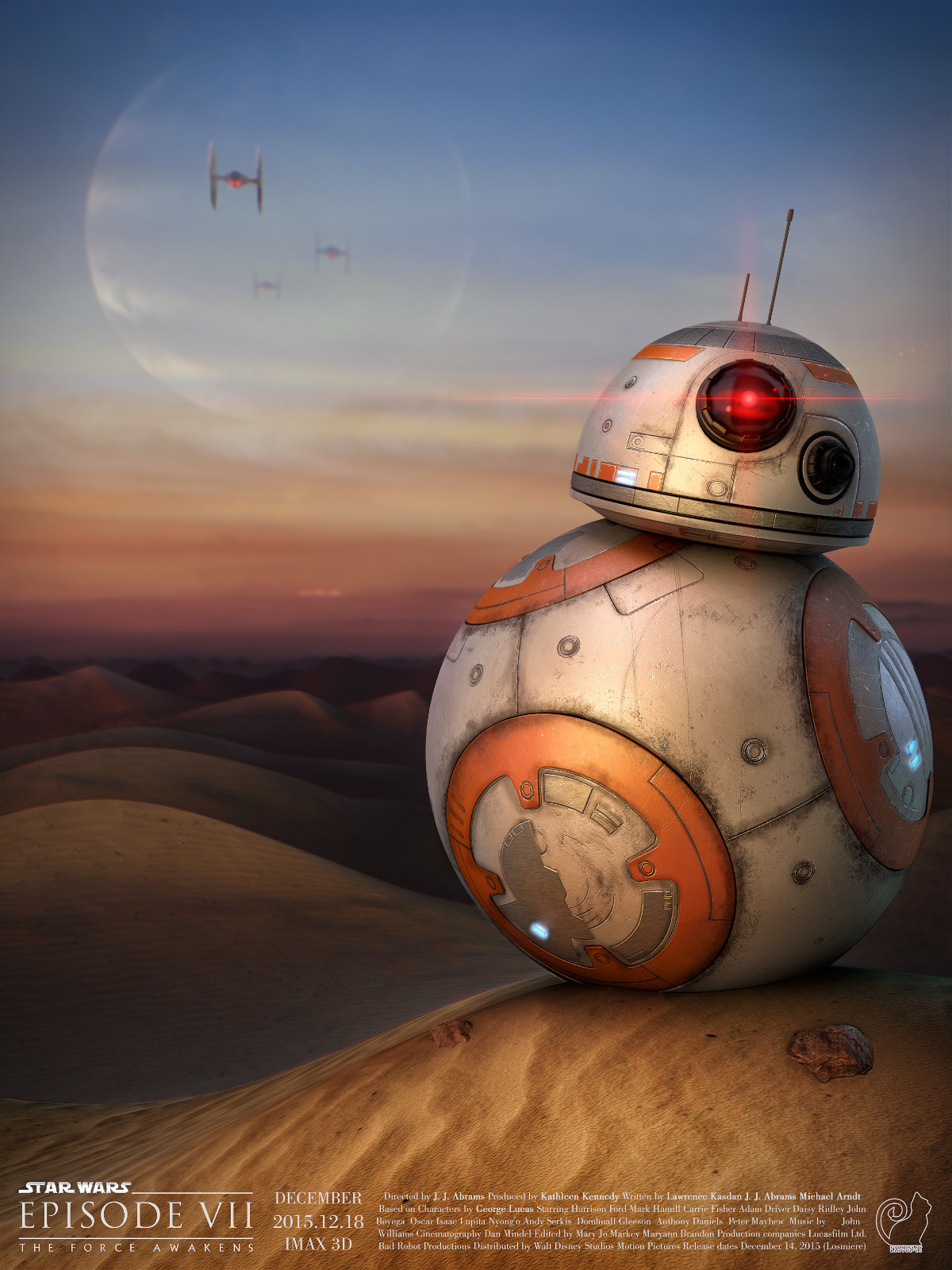The image is a color illustration in portrait orientation, featuring a close-up of the droid BB-8 from Star Wars Episode VII: The Force Awakens. The poster has the dimensions of a sheet of paper and prominently displays BB-8, positioned on the right side. BB-8, a spherical robot made of silver metal with orange disks and plates around its circular body, has a half-dome-shaped head with a red light on top, which casts a warm glow over its upper section. The droid also has an antenna sticking out from its head.

Set in a desert environment, BB-8 rests on a dune covered in beige sand, while additional darker dunes stretch out on the left toward the horizon. The background sky, taking up about half of the image, transitions from a dark purple near the horizon to a twilight blue, with the sun casting a red hue. Starfighter aircraft can be seen in the distance on the top left, approaching, along with the outline of a large planet.

Text along the bottom of the image includes the Star Wars logo on the bottom left corner, with "Episode VII: The Force Awakens" beneath it. Further details such as "December 2015," "1218 IMAX 3D," and credits for the director JJ Abrams, producer Kathleen Kennedy, and writers Lawrence Kasdan, JJ Abrams, and Michael Arndt, based on characters by George Lucas, are also included. A white cat logo is present in the bottom right corner.